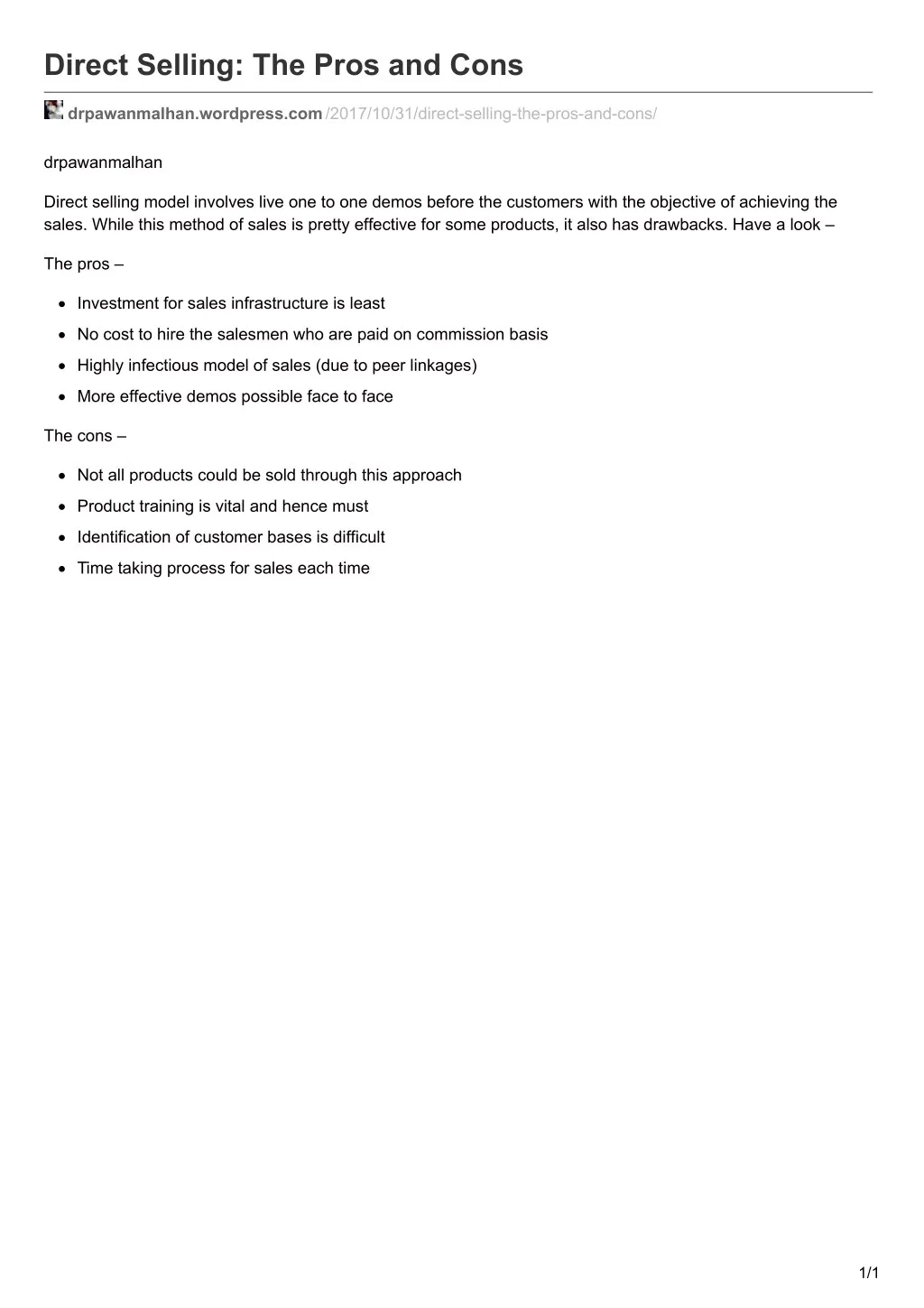Screenshot of a Document Discussing Direct Selling

This image is a screenshot of a single-page document focused on the topic of direct selling. The title, "Direct Selling: The Pros and Cons," is prominently displayed at the top of the page in bold black font. Beneath the title, a thin gray line runs horizontally across the page, separating the header from the body of the text.

On the left side of the page, there is a very small square profile photo. To the right of this profile photo, the following website URL is listed: "drpaulinmalhan.wordpress.com/2017/10/31/direct-selling-the-pros-and-cons/". Below this URL, the text begins with a brief introduction: 
"Dr. Paulin Malhan explains that the direct selling model involves live one-to-one demos before customers with the objective of achieving sales. While this method of sales is quite effective for some products, it also has its drawbacks. Have a look."

The section is then divided into two main parts: "The Pros" and "The Cons".

**The Pros:**
- Investment for sales infrastructure is minimal.
- No cost to hire salesmen, who are paid on a commission basis.
- Highly effective model due to peer linkages.
- More effective demos are possible face-to-face.

**The Cons:**
- Not all products can be sold through this approach.
- Product training is vital and thus necessary.
- Identification of customer bases is difficult.
- The sales process is time-consuming each time.